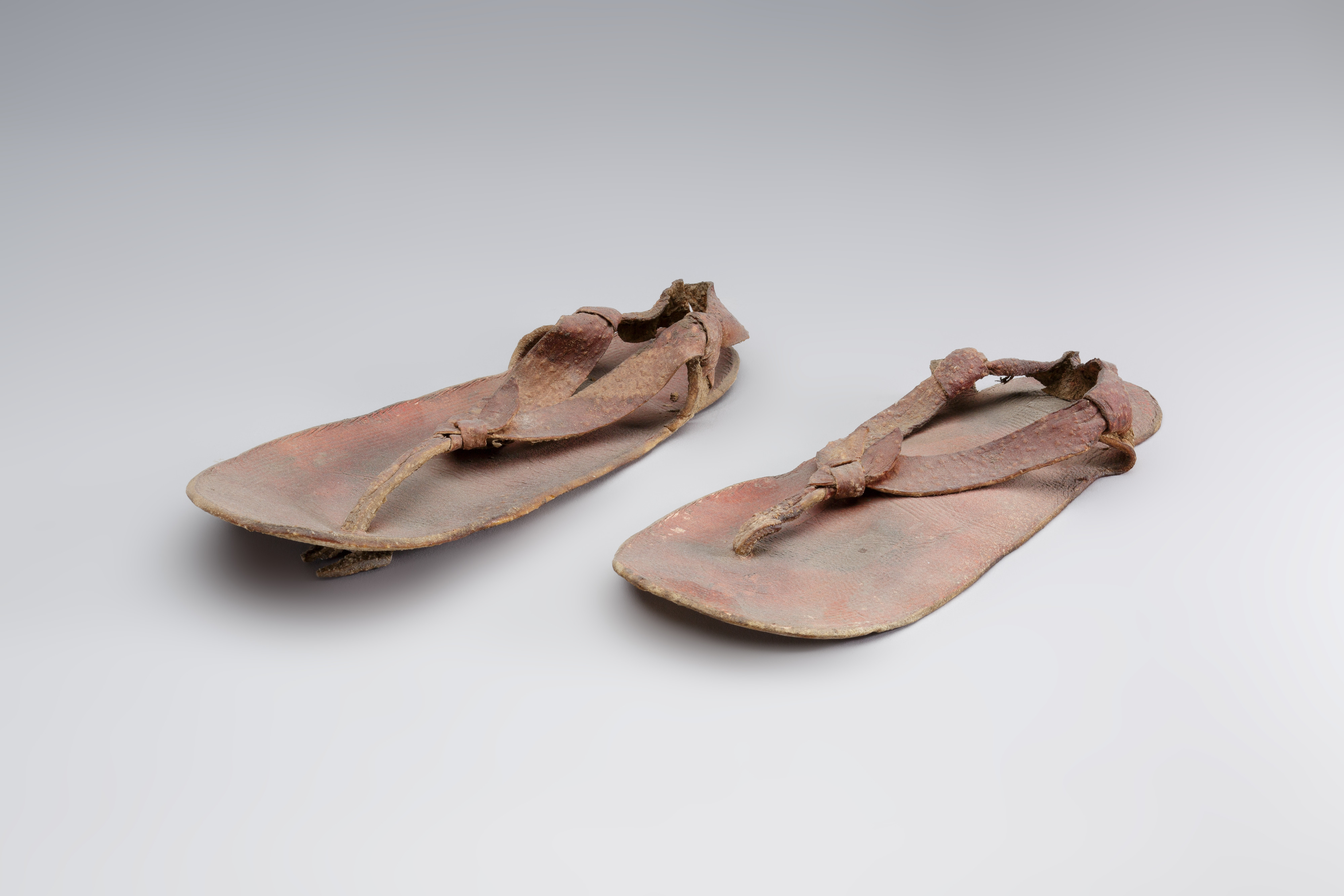On a light gray, slightly gradient background, a pair of ancient, vintage sandals is displayed. These sandals, appearing very old and weathered, are a dull, dusty burgundy color. Made from leather, they feature toe straps fashioned from rope that weave between the big toe and other toes, securing the sandals around the back of the ankle. The soles are notably flat, offering almost no padding, and are laced with strings that hold the worn-out straps in place. Heavy shadows cast beneath emphasize the texture and age of these potentially Native American relics.